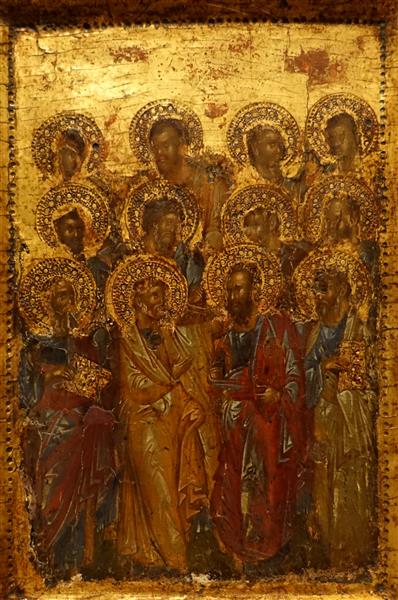This image is a photograph of a gold-hued religious painting, likely depicting Apostles from the Bible. The background features a richly gilded, perhaps bronze-tinged surface with a brilliant, reflective quality. The painting is structured in a rectangular format, showcasing three horizontal rows and four vertical columns of figures, making a total of twelve individuals. Each figure is adorned with a distinct halo, characterized by ruffled, golden edges that surround their heads. These figures appear solemn, wearing various colored robes—some in red and gold— with a few depicted holding books. The men's faces, some bearded and a couple bald, are serious and contemplative as they look in various directions, though none are gesticulating. The painting exhibits an antiquated charm with visible signs of age, such as cracks and a slightly blurred detailing. The entire scene is framed by an intricately bejeweled edge, enhancing its sacred and venerable appearance.